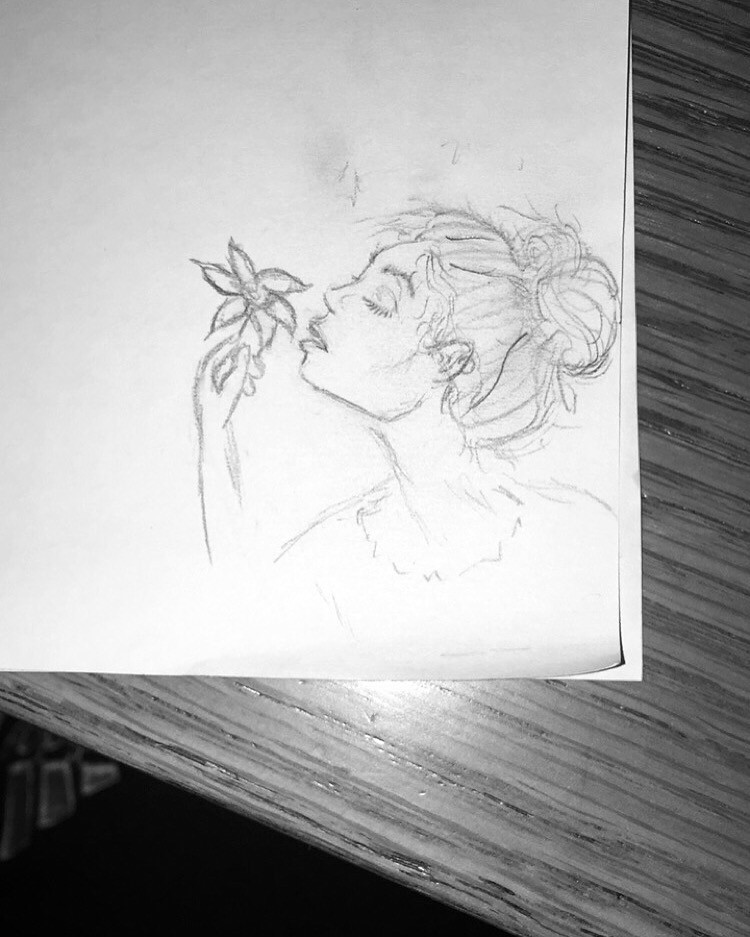This image captures a detailed sketch on a large sketch pad, occupying the left portion of the frame and descending about 75% of the way down. The composition of the photograph is taken from an overhead angle, revealing a portion of a grayish wooden tabletop in the background. The drawing itself portrays a woman with her eyes closed, delicately holding a flower close to her face as if she is savoring its fragrance. Her hair is styled up in a bun, adding a touch of elegance to her serene expression. The textured strokes and careful detailing of the sketch highlight the artist's skill in capturing both the subject's poise and the tranquil moment.